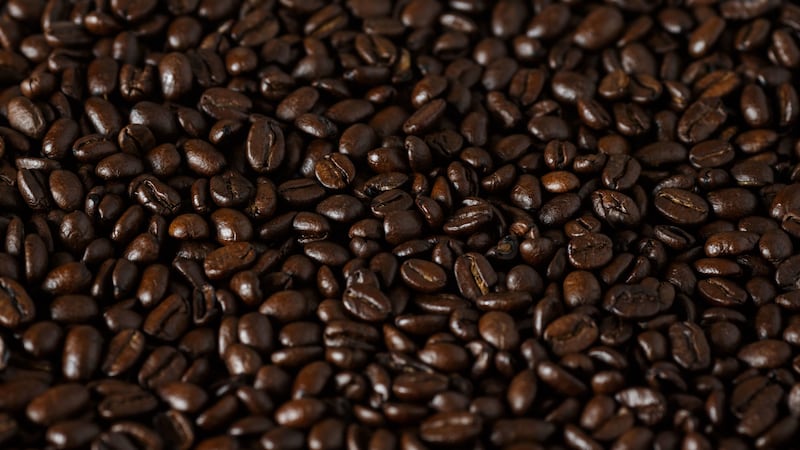This is a highly detailed, very zoomed-in rectangular image depicting an impressive pile of dark brown, freshly roasted coffee beans. The composition showcases hundreds, if not thousands, of whole beans densely packed together, creating an almost impenetrable mass of rich, glossy coffee. The beans vary slightly in appearance; while some appear perfectly whole, others seem partially cut or halved, adding texture to the scene. Their shiny surface suggests a dark roast, possibly giving the illusion of wetness. Each bean features a distinctive indented line in the middle, providing a focal point amidst the sea of uniformity. The image hints at a lower central area with slightly blurred corners, suggesting layers upon layers of beans similar to those found in bulk coffee bins at supermarkets. This vibrant array encapsulates the essence of coffee readiness, poised for grinding or brewing.